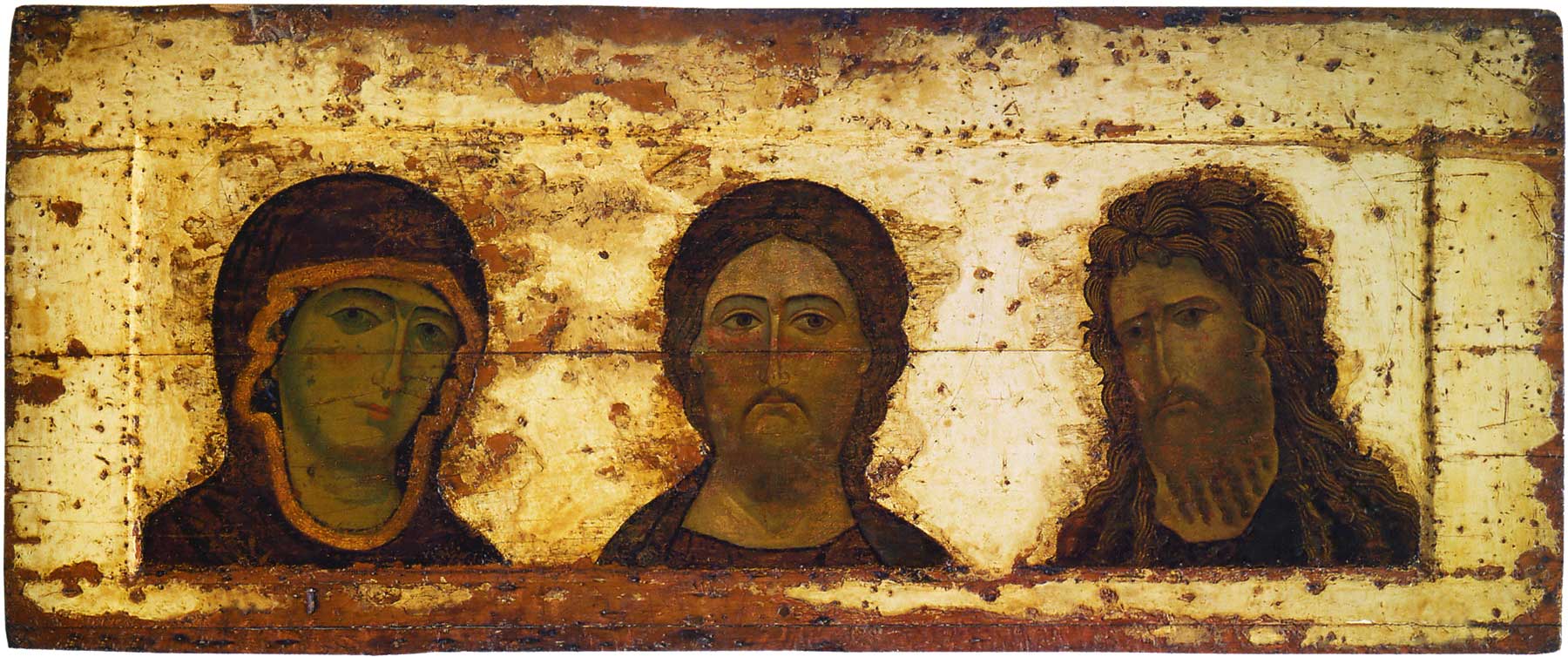The image showcases an ancient piece of art, possibly on a rectangular wooden plank or a piece of metal, evident from its rustic and stained appearance with rusty edges. At the center of this artwork are three human figures depicted from the head and shoulders, all facing forward and appearing somber. On the left, a likely female figure is draped in a dark red hood and gown with an orange trim, featuring a unibrow, a long thin nose, and small pink lips. In the middle stands a figure reminiscent of Jesus, clad in dark robes, with brown hair and a thin mustache, noticeably frowning. The figure on the far right has long, thick wavy hair and a full wavy beard, wearing a black tunic. The background is rustic with brown splatters, enhancing the artwork's aged look, and there is no visible text in the image. The palette includes subdued tones of white, yellow, red, brown, and gray, reinforcing its historic and artistic feel.